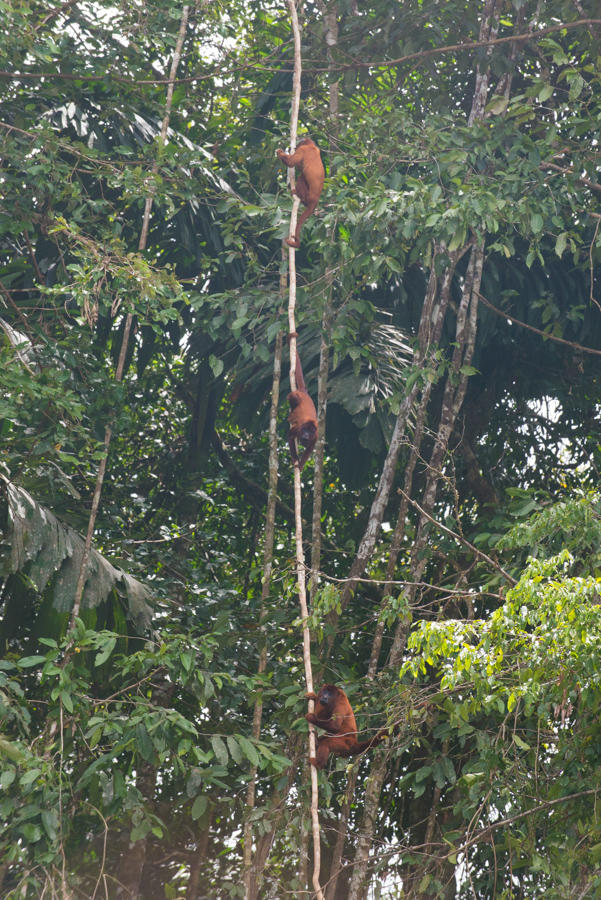The image captures an outdoor scene in a dense, tropical jungle bursting with verdant foliage. Towering trees with thin trunks reach up so high that they almost entirely block the sky, though patches of blue peek through the thick canopy. Amongst the myriad of green leaves, some trees have long, vine-like branches hanging down. Three monkeys, possibly baboons with brown coats and gray faces accentuated by darker patches around their eyes, are climbing these trees. Two seem to be ascending, while one in the middle appears to be descending, using its tail for support. The jungle is so thick that details of the sky are minimal, making it clear that the image focuses on the rich, leafy environment and the playful, agile primates navigating their arboreal playground.